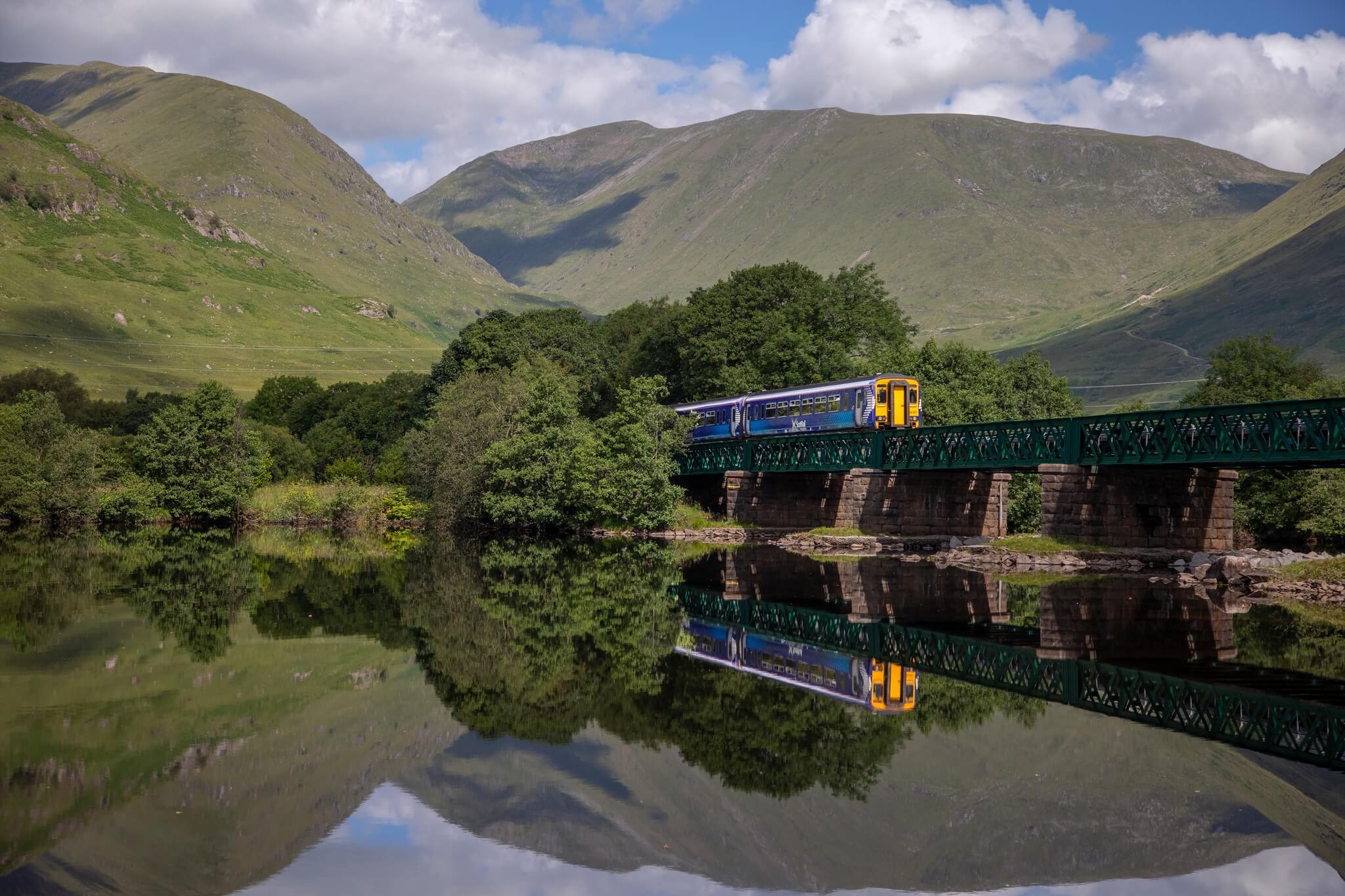This striking daytime photograph captures a picturesque scene of a blue train, accented with a yellow engine, traveling atop a dark green iron railway bridge. The bridge is supported by robust stone columns, and spans a calm, reflective body of water that mirrors the entire scene beautifully. Dominating the mid-ground are large green hills, with an expansive green mountain graced by the shadowy outlines of clouds in the background. The serene landscape is peppered with lush greenery, large trees, and scattered brown patches of land and streets. The clear, bright blue sky adorned with white clouds enhances the tranquil natural setting, reflecting vividly in the tranquil waters below.